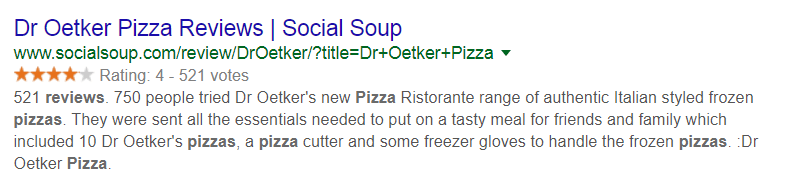This image captures a screenshot of a search result for Dr. Oetker pizza reviews from the website Social Soup. At the top, the title "Dr. Oetker Pizza Reviews" is displayed in blue text. Below, the URL "www.socialsoup.com/review?title=dr+oetker+pizza" appears in green. An arrow pointing downwards is also visible.

The review highlights that Dr. Oetker's pizza has received an aggregate rating of four out of five stars, based on 521 votes. The text reveals that 750 people tried Dr. Oetker's new range of authentic Italian-style frozen pizzas. These participants were provided with all the essentials to host a delightful meal for friends and family, which included ten Dr. Oetker pizzas, a pizza cutter, and freezer gloves to handle the frozen pizzas. The entire background of the image is plain white.